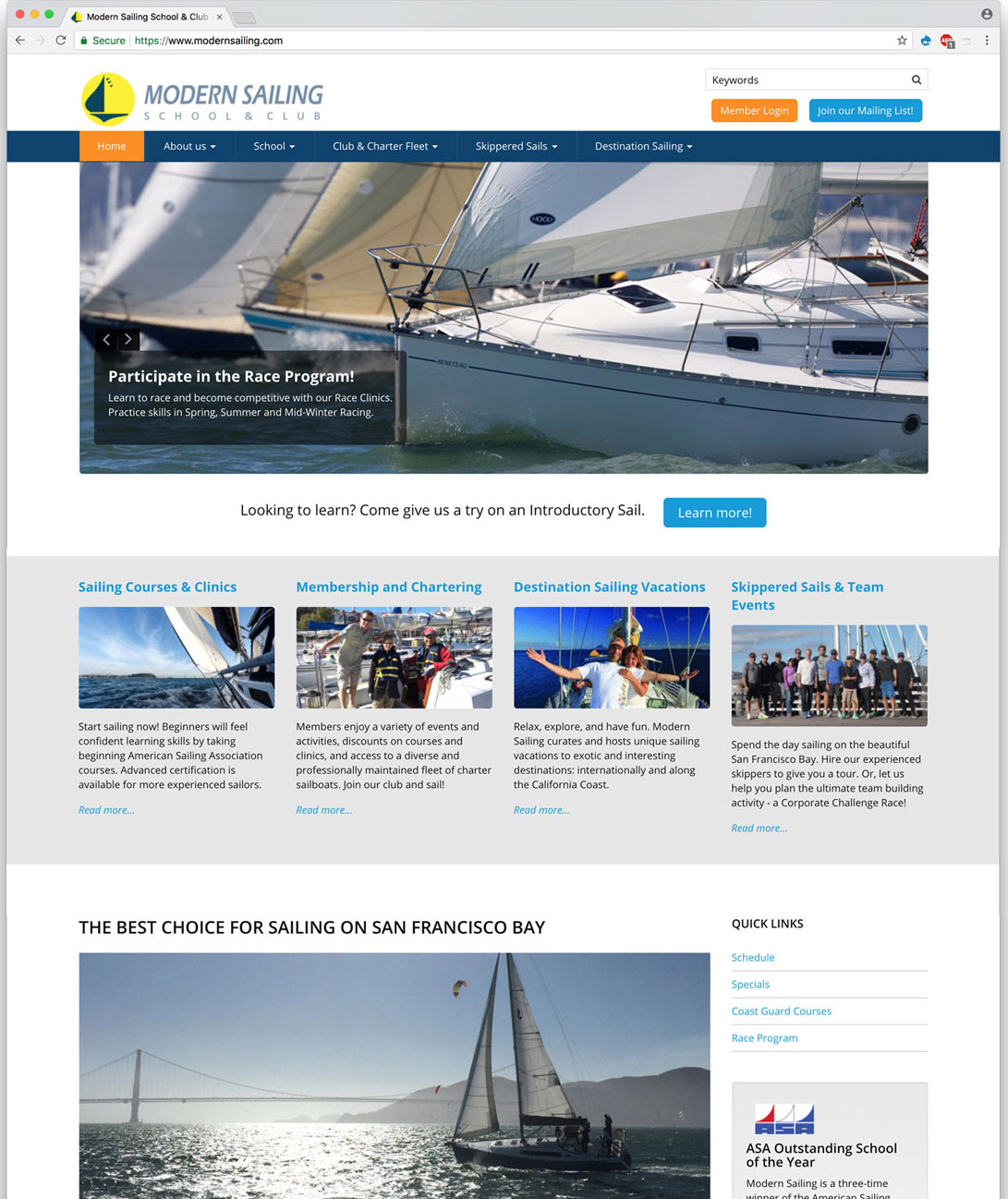This detailed caption describes the various elements visible in an image taken from the Modern Sailing School and Club's website:

---

The image is a screenshot from Modern Sailing School and Club’s official website, ModernSailing.com. At the top, the website's header features the navigation options, including "Home" in orange, followed by "About Us," "School," "Club and Charter Fleet," "Skippered Sails," and "Destination Sailing." On the top right, there are options for "Member Login" in orange and "Join Our Mailing List" in light royal blue.

Prominently displayed at the center of the header is a yellow circular logo with a deep blue sailboat inside. Below the navigation bar, the webpage highlights its offerings with vibrant images and descriptive text. 

Foregrounded is a photo of three sailboats, close to each other on the water, suggesting they might be either docked or sailing in proximity. Accompanying this visual, there is a prompt reading, "Participate in the Race Program," followed by the invitation, "Learn to race and become competitive with our race clinics. Practice skills in spring, summer, and midwinter racing."

Further down, an introductory offer encourages visitors with "Looking to learn? Come give us a try on an introductory sail." The page includes additional images of sailboats and people engaging in sailing activities, alongside informative paragraphs aimed at prospective members.

---